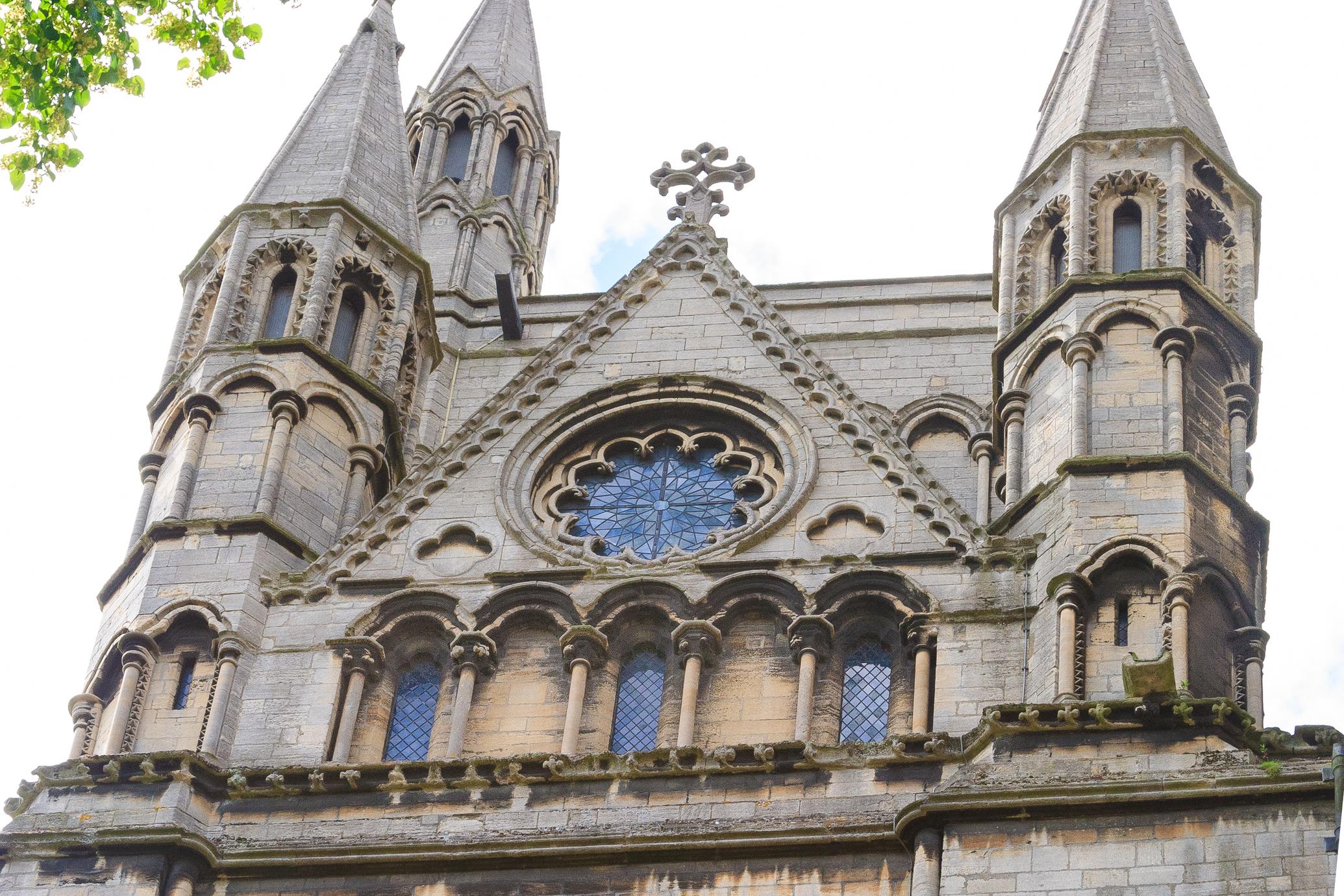The image captures an ornate, older-style church or cathedral, viewed from a low angle that emphasizes its towering structure. The church is constructed from light brown and gray bricks, suggesting a harmonious blend of colors, and exhibits impressive architectural details. Dominating the scene are three tall, peaked steeples, each with a distinct pointed design. The central steeple features a large, circular flower-shaped stained glass window, flanked below by three smaller oval-shaped stained glass windows, creating a striking focal point. At the pinnacle of the middle steeple sits a Celtic cross, adding to the church's gothic aesthetic.

The right side of the frame reveals a tree, with leaves and branches reaching into the shot, while another tree is slightly visible in the left-hand corner. Above, the sky is predominantly clear with patches of clouds, allowing ample sunlight to illuminate the building, casting soft shadows. Despite the building displaying slight signs of aging and dirt, its overall condition appears fairly good, and it retains an inviting, warm appearance. Small water gutters are observed along the edges, hinting at functional elements aimed at preserving the church. The image does not contain any text, ensuring that the focus remains entirely on the intricate details and grandeur of the cathedral.